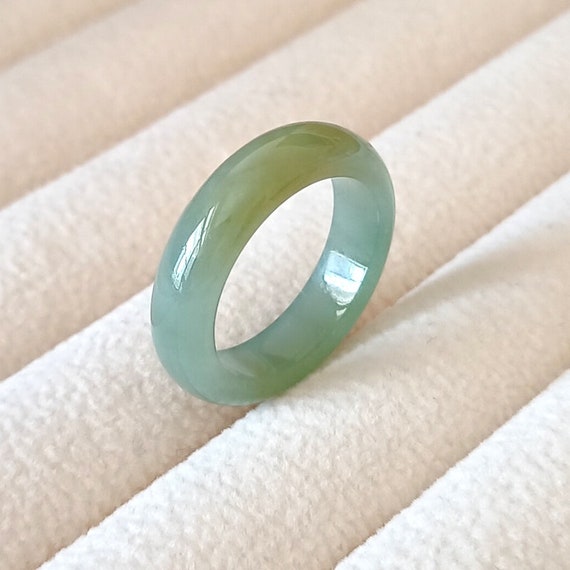The image is an up-close view of the ring section inside a cream-colored jewelry box designed with several round, cushioned areas for placing rings. At the center of the image, a thick jade ring rests vertically on the padding. The highly polished jade ring exhibits various shades of green, including a light green on the sides and a more intense green on the top, along with brownish yellow or golden hues near the top. Its surface reflects a window both on the top and the inner side, emphasizing its shiny, polished texture.